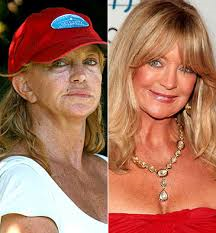In this collage, the left photograph features a woman with golden blonde hair, wearing a white shirt and a red cap adorned with a blue ellipse on the front. She has dark circles under her blue eyes and appears somewhat sunburnt. Her hair is pulled back, and she is gazing off to the left. The right photograph displays the same woman, elegantly dressed in a red outfit, accessorized with a prominent gemstone necklace that drops down in front, paired with matching earrings. The background of the collage is white with some blue text visible. The woman, who resembles Goldie Hawn, ties both photos together with her distinctive blonde hair and striking blue eyes.